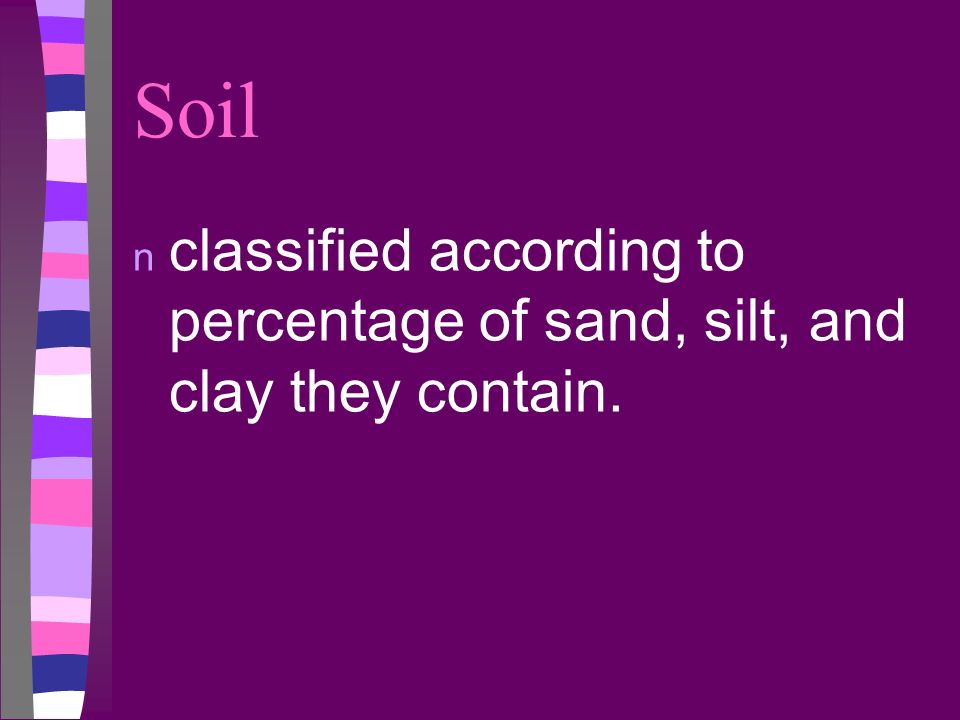This image features a PowerPoint slide, predominantly showcasing text with no particular objects. The background is a light purple or violet. On the left-hand side, there are various colorful rectangles and squares, forming a vertical spectrum of shades, including dark purple, pink, light purple, dark pink, dark blue, yellow, brown, lavender, and white, set against a grayish background. In the top left corner, the word "soil" is highlighted in pink. Below it, the letter "N," indicating "noun," is displayed in a purplish-blue hue. The main text in white reads, "classified according to percentage of sand, silt, and clay they contain." The style of this slide suggests it is intended for educational use, offering a vibrant and visually engaging learning tool.